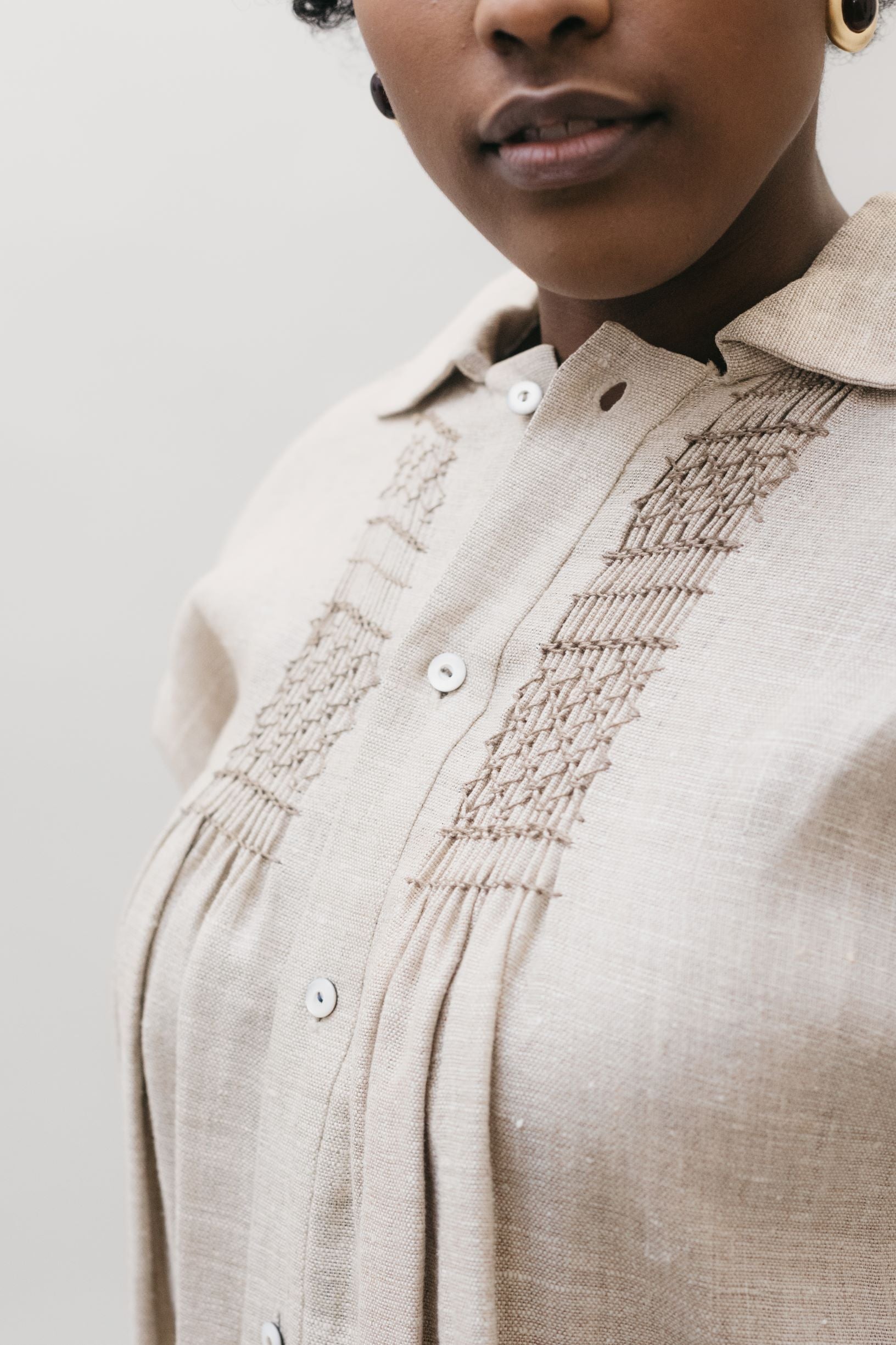This image is a close-up photograph of an African-American woman, showing her from the nose down with her eyes and the top of her head cropped out. The woman has a small amount of black, curly hair visible at the top edge of the frame, and she is half-smiling while looking toward the camera. She wears a pair of earrings that are just below her short hair. Her attire is the main focal point: a simple yet elegantly designed beige or light tan linen shirt. The shirt features white buttons, almost matching the shirt’s color, running vertically down the front. It has a delicate vertical texture near the buttons and subtle embroidery or applique along with two side pleats at the bust line. The fabric appears softly gathered near the buttons, providing a form-fitting design at the top and a fuller, pleated appearance below. The background is plain, a solid white wall that enhances the focus on the woman and her textured, carefully designed shirt.